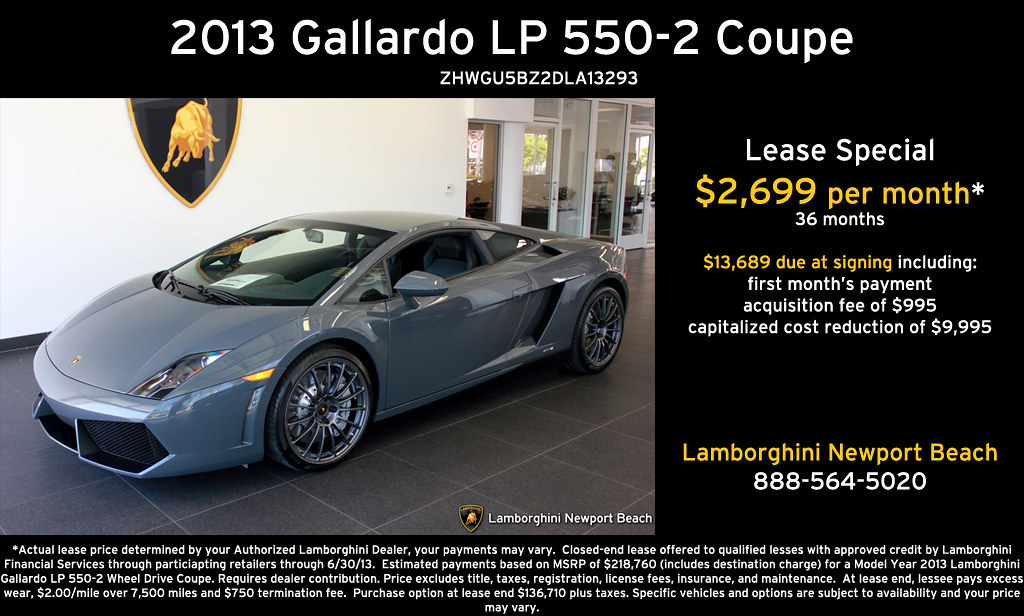This is an advertisement for a 2013 Lamborghini Gallardo LP 550-2 Coupe. Set against a black background with white text, the ad prominently features the car's model name with its VIN number beneath it. On the right side, the text advertises a lease special with "Lease Special" in white and "$2,699 per month*" in yellow, followed by "36 months" in white. Further details include "$13,689 due at signing, including first month's payment, acquisition fee of $995, capitalized cost reduction of $9,995" in smaller white text. Additionally, the dealership's name "Lamborghini Newport Beach" is in yellow with their contact number "888-564-5020" in white below it.

On the left side of the image is a sleek, gray Lamborghini 550-2 Coupe showcased inside a dealership. The showroom's white wall features a gold Lamborghini insignia above the vehicle. In the background, the dealership's doors are visible. The image emphasizes the car's elegant design in a standing position, highlighting its luxurious and sophisticated appearance. Smaller white text at the bottom of the ad provides further lease terms and conditions.